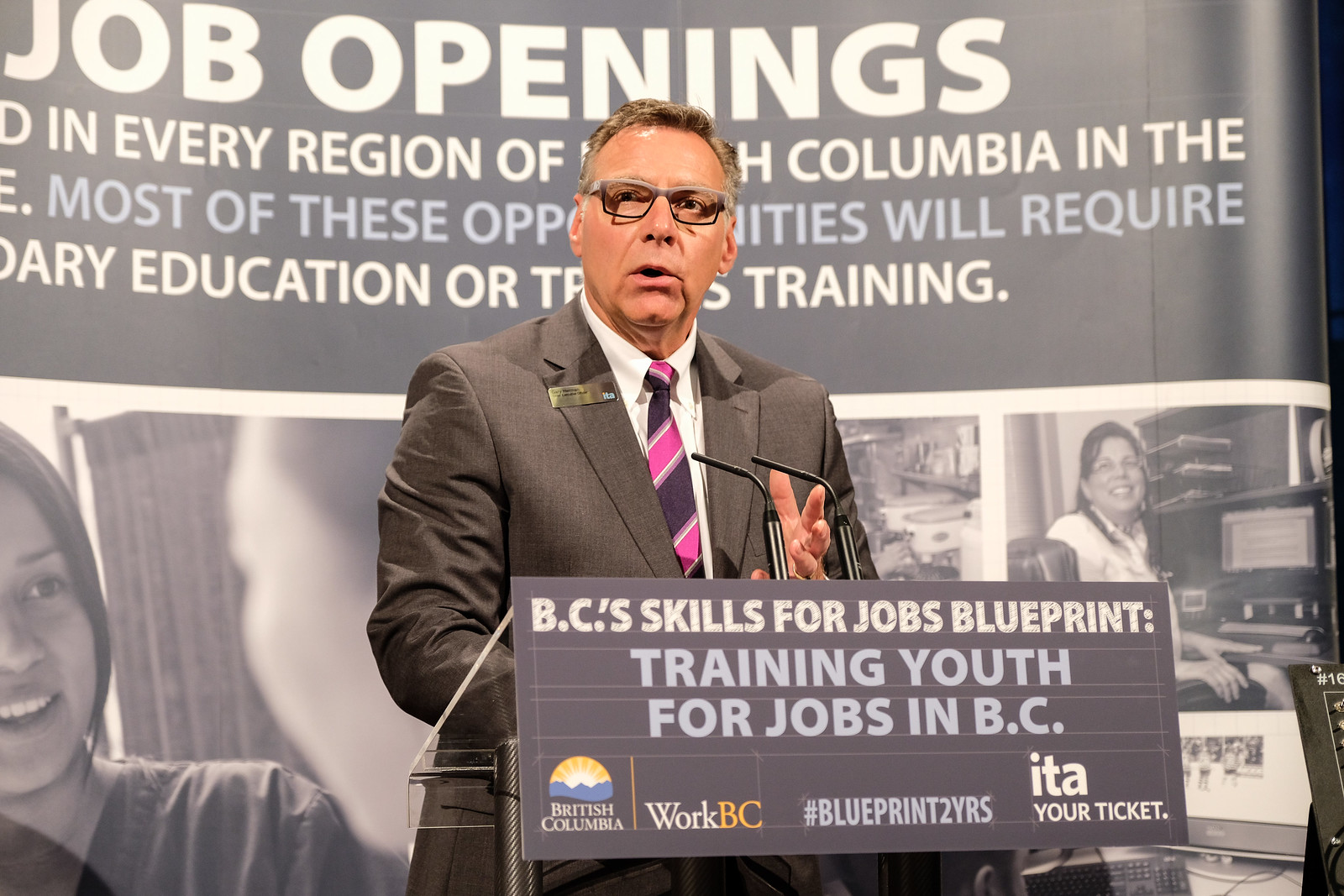In the image, a middle-aged man with salt and pepper hair stands at a podium, positioned slightly to the right of center. He is delivering a presentation at an indoor event focused on job training opportunities. The man is dressed in a dark grey suit, a white button-down shirt, and a pink and purple striped tie. He also wears prescription glasses with frames that fade from light grey at the top to black at the bottom and has a metallic name tag on his lapel.

The podium features multiple inscriptions; prominently, it reads, "BC Skills for Jobs Blueprint," accompanied by phrases such as "Training youth for jobs in BC," "British Columbia," "Work BC," "#Blueprint2Years," and "ITA, your ticket." Behind the speaker is a poster with text and graphics, mentioning "job openings in every region" and noting that "most of these opportunities will require education or training."

The scene is accented with a variety of colors including tans for the man's skin, pink and purple for his tie, and an assortment of blues, blacks, yellows, and whites in the background graphics and signage. The setting suggests a formal presentation aimed at discussing job training and employment opportunities within British Columbia.